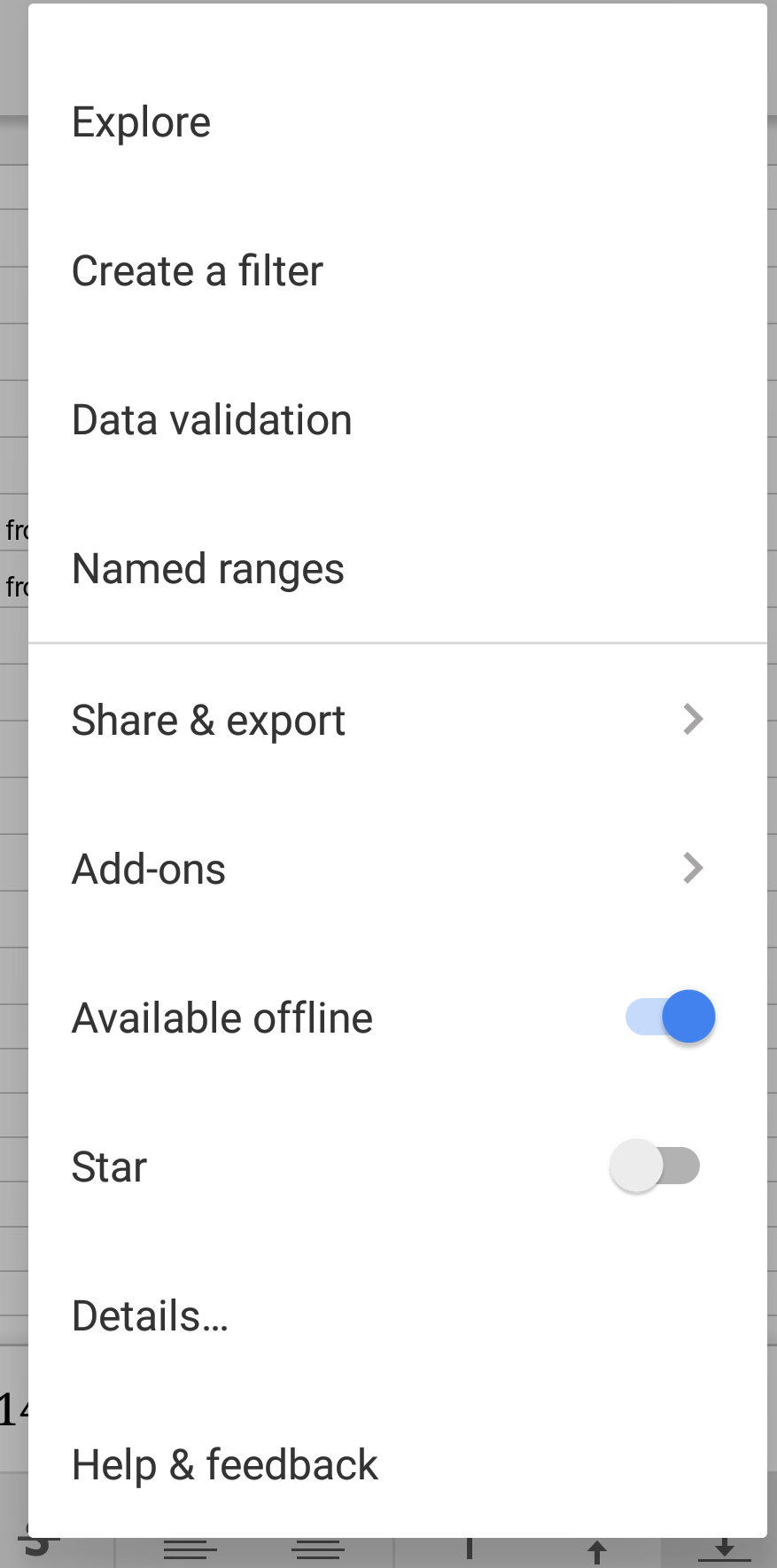The image showcases a drop-down menu that mimics the interface typically seen when right-clicking with a mouse. This menu displays several options arranged vertically, each text written in black. The options listed, from top to bottom, include: "Explore," "Create a Filter," "Data Validation," "Named Ranges," "Share and Export," "Add-ons," "Available Offline," "Star," "Details," and "Help and Feedback."

Notably, both "Available Offline" and "Star" feature toggle bars. When activated, these toggles appear blue; when deactivated, they are black and white. The "Share and Export" and "Add-ons" options have accompanying arrows, indicating the presence of additional submenus.

Dominating the entirety of the image, the drop-down menu is set against a background that resembles an Excel spreadsheet. The menu itself is framed by a gray outline on the left and bottom edges, likely emphasizing its boundaries within the larger context of the spreadsheet interface.